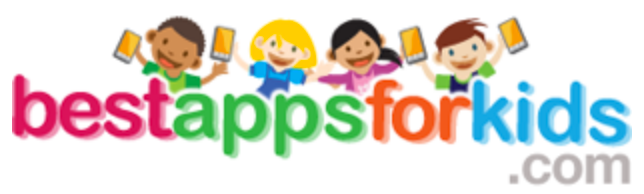The logo for BestAppsforKids.com is displayed prominently against a clean white background. The text is colorfully arranged, with "Best" in purple, "Apps" in green, "for" in orange, "kids" in blue, and "dot com" in gray. Above the text, there are illustrations of four excited children, each holding a smartphone. The children have different hair colors—one with brown hair, one with blonde hair, another with black hair, and another also with brown hair—and they each wear a brightly colored shirt: green, blue, purple, and a mix of blue and green. The design resembles a webpage or digital advertisement, likely representing a company that provides apps targeted towards children. The enthusiastic expressions on the children's faces suggest an engaging and fun experience, hinting at the entertaining and educational nature of the apps available on the website.